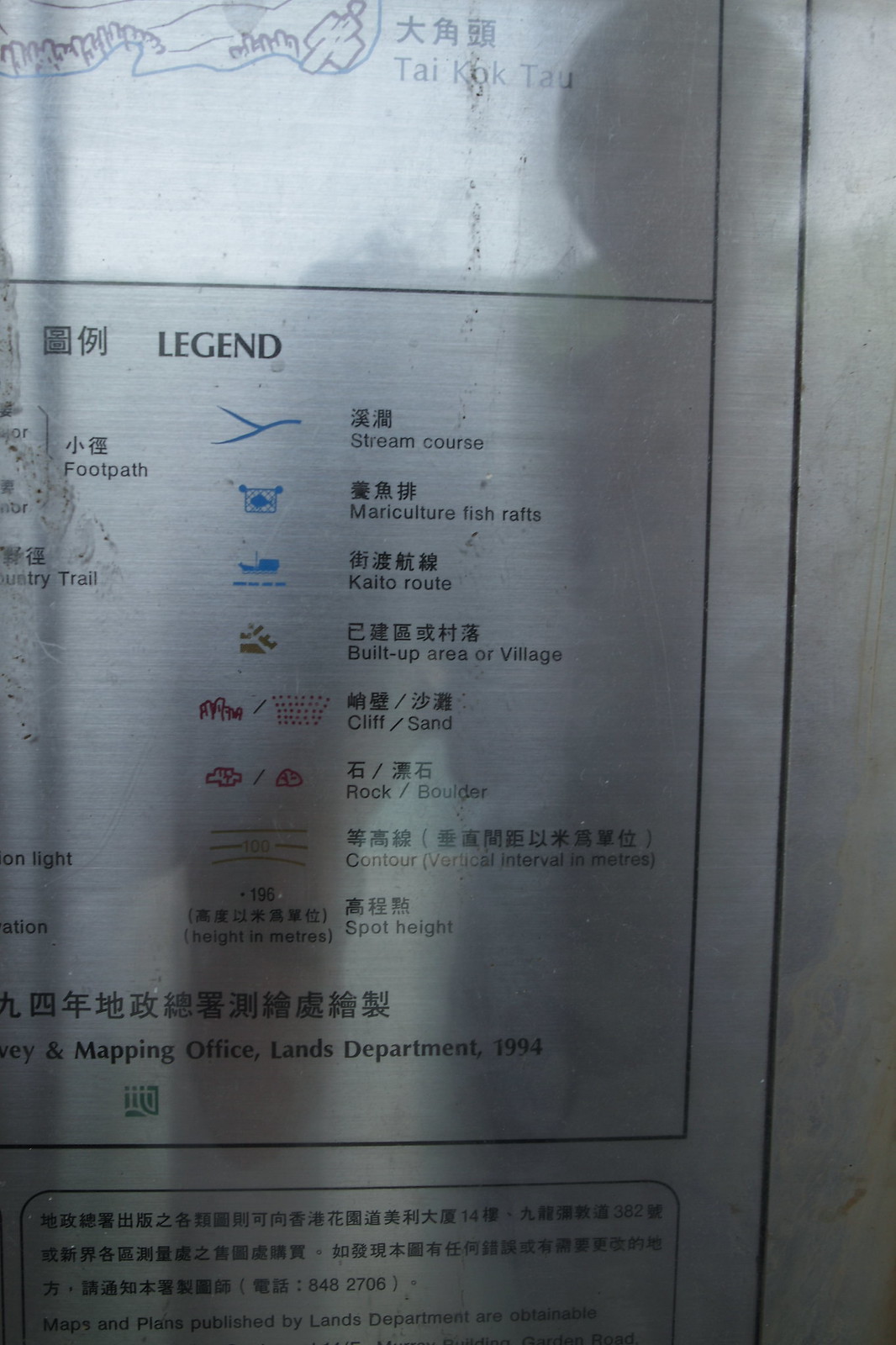The image captures a legend of a map, likely a tourist attraction or city map, predominantly in an Asian language, potentially Chinese or Japanese. The legend, titled "Tai Kok Tao" with accompanying Asian characters, details various map features such as footpaths, country trails, stream courses, mariculture fish rafts, kaitou routes, built-up areas or villages, cliffs and sands, rock boulders, contours, vertical intervals in meters, heights in meters, and spot heights. The map legend, protected by glass, bears a silhouette of the person who took the photo. The text indicates it was created by the Survey and Mapping Office of the Lands Department in 1994. Additionally, the map mentions that plans published by the Lands Department are obtainable, although this part is partially cropped out. The material of the map appears to be plastic with horizontal lines, displayed in a somewhat dim but light environment. The text visible includes the number 8482706 and multiple Asian language characters.